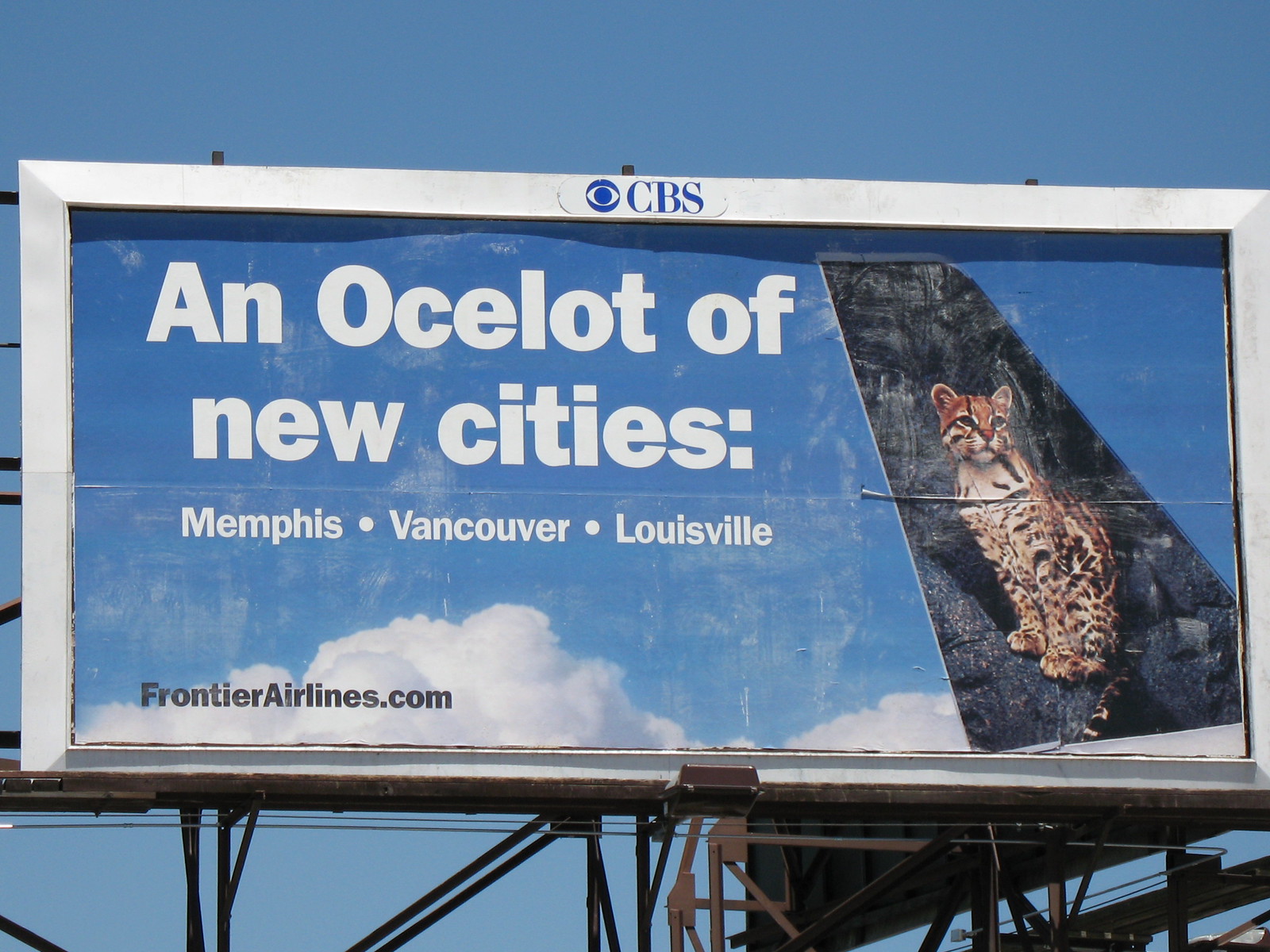The photograph captured in vibrant color and set against a pristine, cloudless blue sky depicts a striking outdoor billboard. The billboard's structure is composed of a lattice of intersecting metal posts, supporting the main display. At the top of the billboard, encased in a silver trim, is the iconic "CBS" lettering alongside the CBS eye logo.

The main advertisement on the billboard features promotional text that reads, "Discover a New City: Memphis, Vancouver, Louisville." Positioned in the bottom left-hand corner in bold black letters is the website "FrontierAirlines.com." Meanwhile, in the bottom right-hand corner of the billboard, there is a detailed image of an airplane wing. Adorning the wing is a lifelike depiction of a cheetah, artistically positioned to appear as though it is perched on stylized, stone-like surfaces drawn onto the wing. The composition and design elements come together to create a visually engaging and meticulously detailed advertisement.